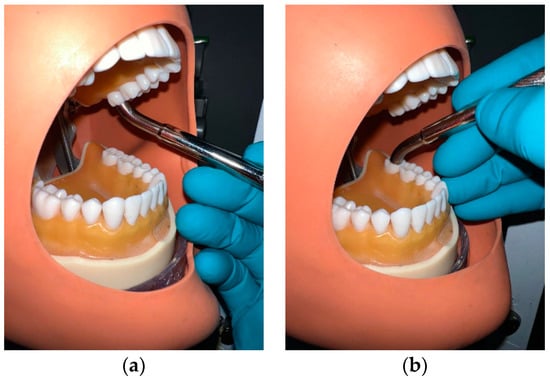The series consists of two side-by-side photographs labeled A on the left and B on the right. Both images feature a dental training mannequin with a Caucasian-colored plastic face that lacks distinguishing features like eyes or a nose. The mannequin's mouth is wide open, revealing detailed representations of an upper and lower jaw complete with white plastic teeth and gum lines. In each photo, the gloved hand of a dentist is visible, wearing blue surgical gloves and holding a silver dental tool. In the left image (A), the tool is in contact with the upper teeth, specifically targeting the back molar, while in the right image (B), the focus shifts to the lower teeth’s back molar. These photos illustrate a dental training or instructional scenario, likely used for educational purposes in dentistry to demonstrate techniques such as polishing or filling cavities.